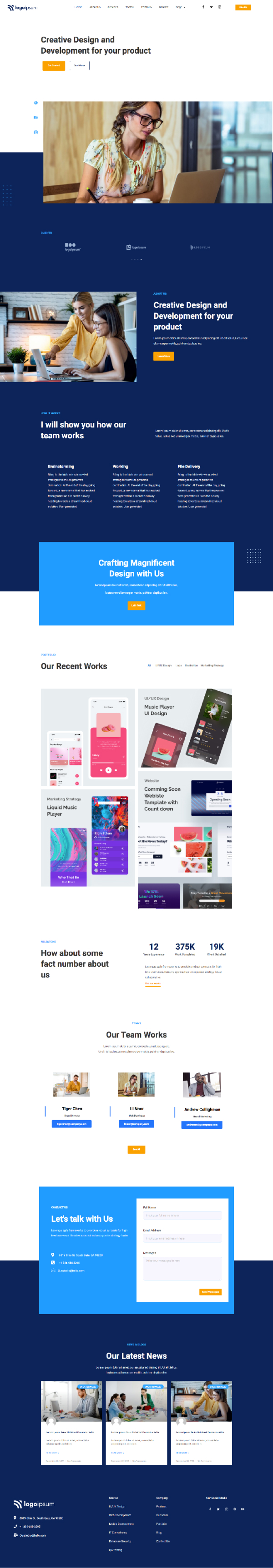The image is quite blurry, making it difficult to discern specific details. It appears to be a screenshot showcasing several open folders or possibly windows on a computer screen, likely related to office supplies. The top section shows what seems to be various folders, while another section below includes a smaller image of a person looking at computer screens. This suggests a multi-tasking scenario, possibly involving a website or catalog for office essentials such as notebooks, paper, calendars, and other supplies. The overall theme points towards office management tools, with the multiple open screens hinting at a cluttered desktop environment typically associated with administrative tasks.